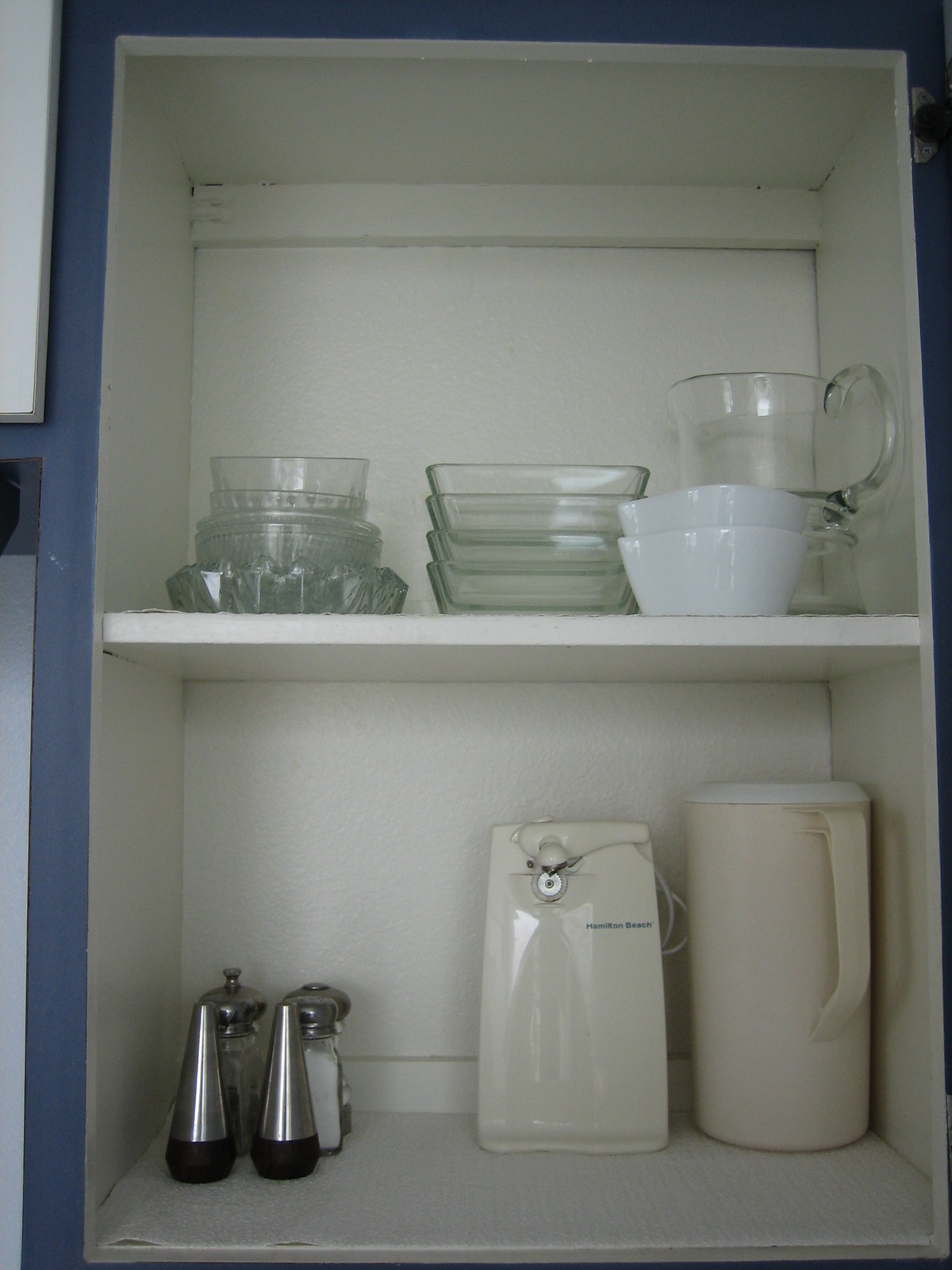This slightly vertical image features two shelves within a built-in hutch-type storage area, likely located in a kitchen. The shelves and the interior of the storage area are painted a pristine white, while the exterior face sports a deep blue with a gray undertone. The cabinets are doorless, revealing the neatly arranged items within.

On the top shelf, a variety of kitchenware is meticulously organized:
- To the left, glassware, condiment dishes, and candy dish-type objects are stacked.
- In the center, there are four square or rectangular glass items which could be bowls or cookware.
- On the right, a pair of white mixing bowls is accompanied by a clear glass measuring cup, notably devoid of any measuring marks.

The lower shelf hosts an assortment of kitchen essentials:
- On the left, there are two pairs of salt and pepper shakers. The front pair is cone-shaped with black bottoms, suggesting they are grinders. Behind them is a more traditional set made of glass with metal screw caps.
- To the right of the shakers sits a tall, likely quart-sized, almond-colored pitcher with a white lid.
- Positioned centrally between the salt and pepper shakers and the pitcher is an electric can opener, also in almond.

The image captures a well-organized kitchen storage area, presenting a blend of utility and aesthetic simplicity.